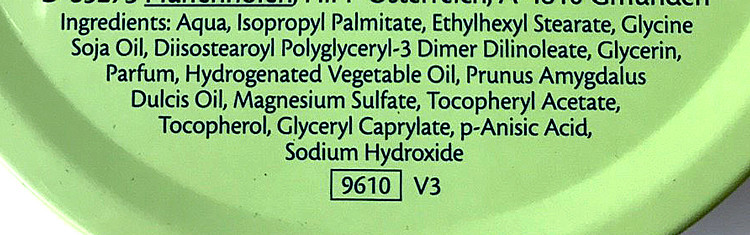This close-up photograph captures a segment of a circular green label, possibly resembling a plate or the lid of a can, from a hair care product or cosmetic cream. The image focuses on the list of ingredients, featuring detailed text that includes aqua, isopropyl palmitate, ethylhexyl stearate, glycine, soja oil, disosteryl, polyglycerol-3, dimer dillinoate, glycerin, parfum, hydrogenated vegetable oil, prunus amygdalus dulcis oil, magnesium sulfate, tocopherol acetate, tocopherol, glycerol caprolate, p-anisic acid, and terminating with sodium hydroxide. Additionally, the label shows "960" inside a square and "V3" adjacent to it. The lime green background and rounded edge frame the text, highlighting the dense and complex ingredient list typical of such products.